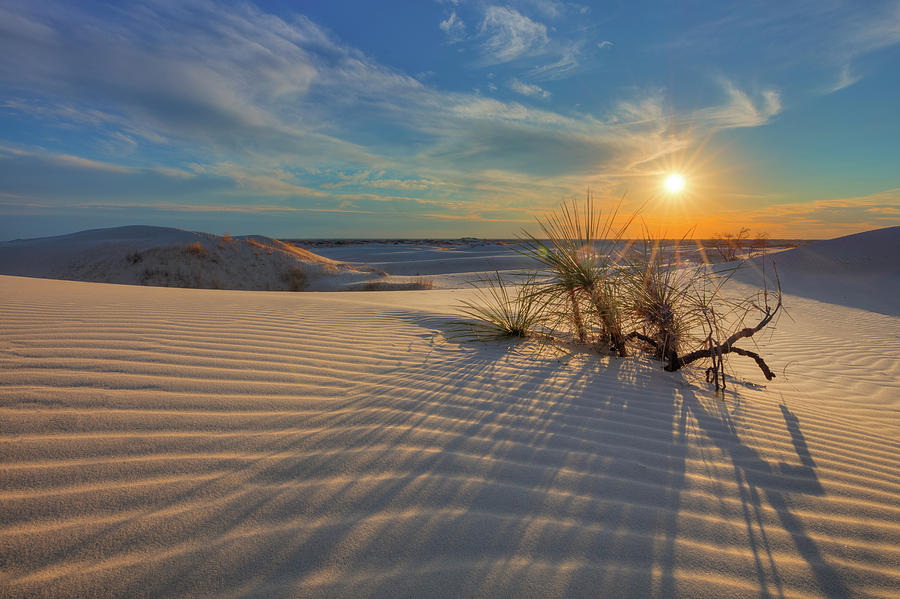In this photograph of a vast desert landscape at sunset, the scene unfolds with rippling sand dunes that stretch endlessly into the horizon, shaped by the persistent wind and marked by intricate ridges and rivets. The sky above transitions from deepening blue to a vibrant orange-yellow near the setting sun, which casts long shadows and lends a golden hue to the terrain. Scattered across the barren expanse are sparse vegetations, including a solitary, small cactus that stands out among the dunes. Wispy clouds swirl gently across the otherwise clear sky, emphasizing the expansive emptiness of the environment. There are no signs of human presence, only the serene and stark beauty of the natural desert, bathed in the warm glow of the fading sunlight.